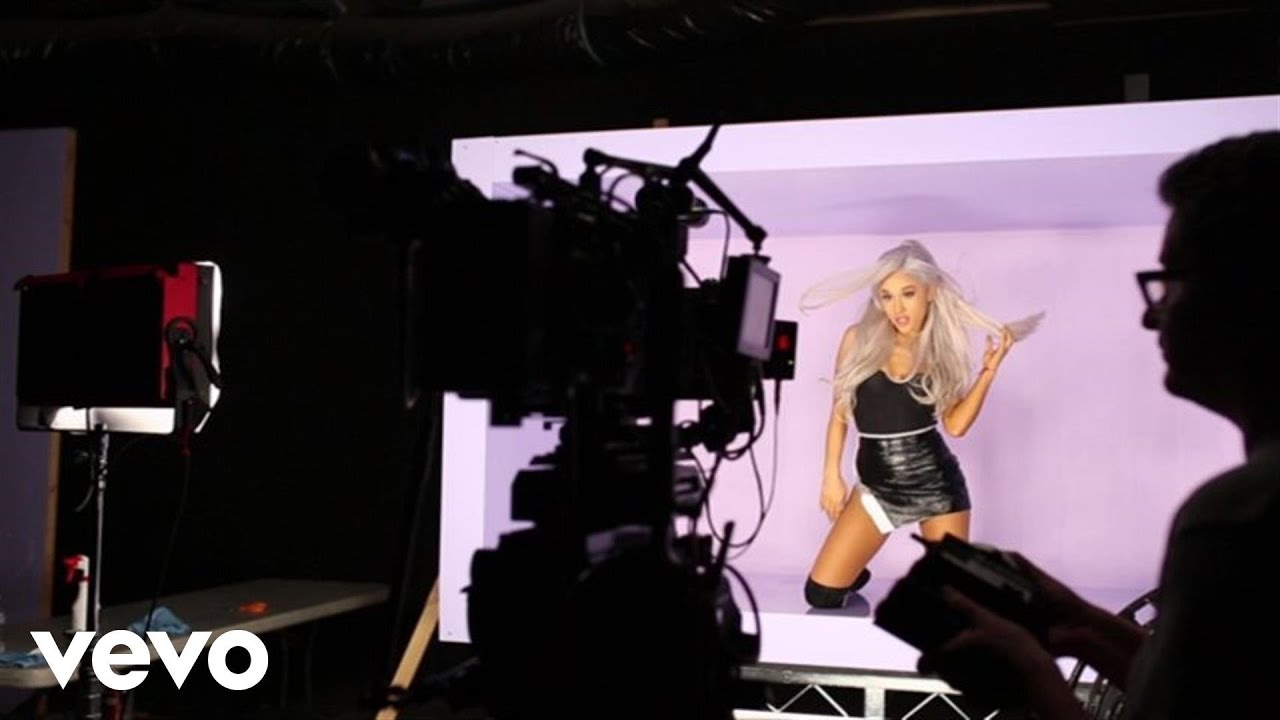The photograph captures a behind-the-scenes moment of an Ariana Grande music video shoot. Set against a light lavender backdrop, Ariana is performing confidently while kneeling in a white box. Her long, almost white platinum blonde hair and her tight black outfit—a skirt and top—stand out vividly. She has a tan complexion, further accentuating her stage presence. To the far right, a man, likely the director, is visible, holding a remote control pointed at one of the high-end cameras arrayed around Ariana. The scene is bathed in intricate lighting, enhancing the visual appeal. At the bottom left of the image, the VEVO logo appears in white, lowercase sans-serif font, marking the association with the popular music channel on YouTube. The image is a glimpse into the meticulous production effort behind Ariana Grande's performance.